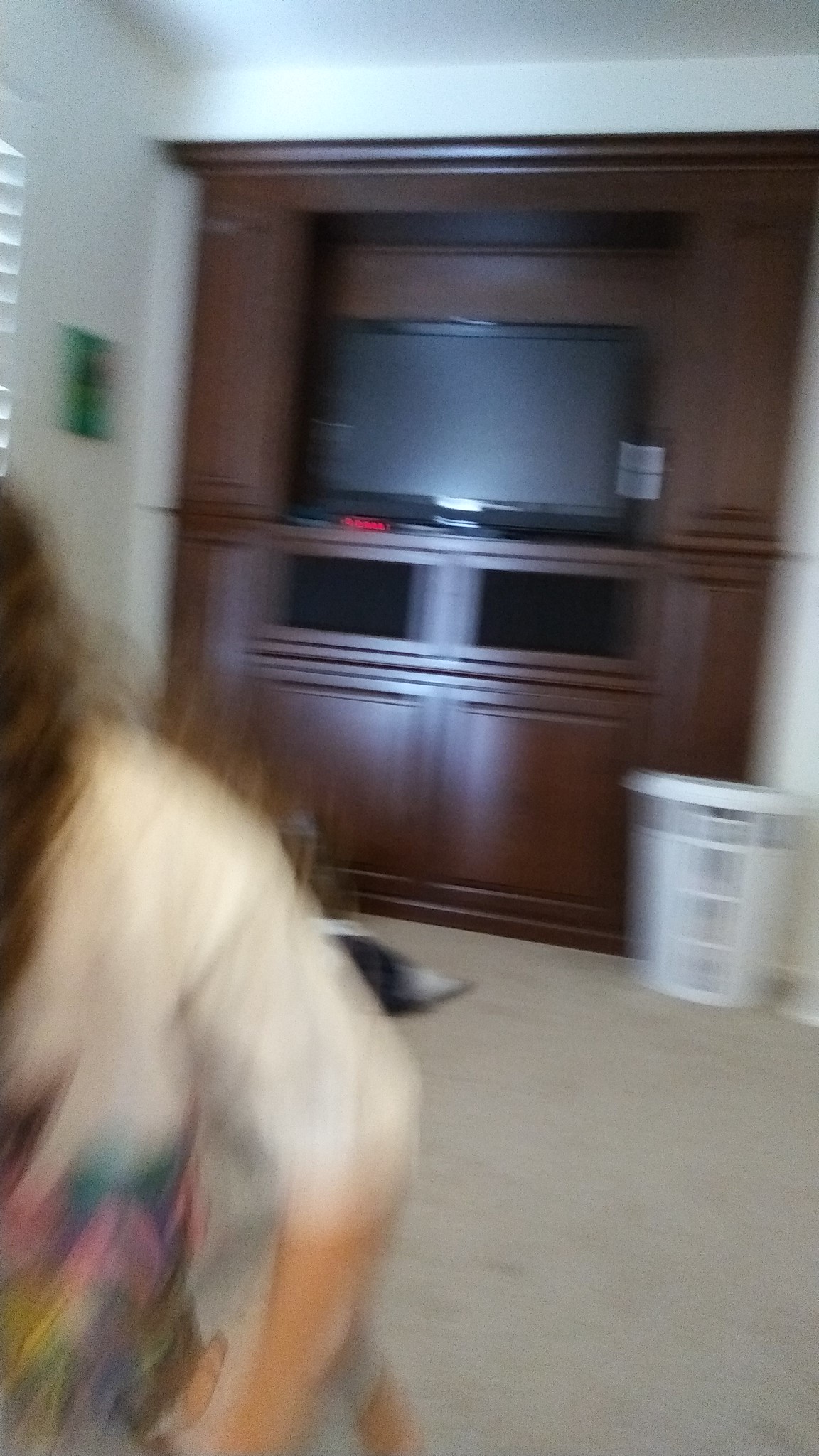Despite being blurry and of low resolution, this image captures a dynamic scene. On the bottom left, a person with brown hair is caught mid-motion, adding to the blurry effect. They are wearing a white shirt, which features a colorful artwork with hints of pink, green, purple, yellow, and brown, though the details of the design are indistinct due to the image quality. In the background, a large, rectangular TV with a black frame is prominently displayed atop a substantial piece of dark brown furniture.